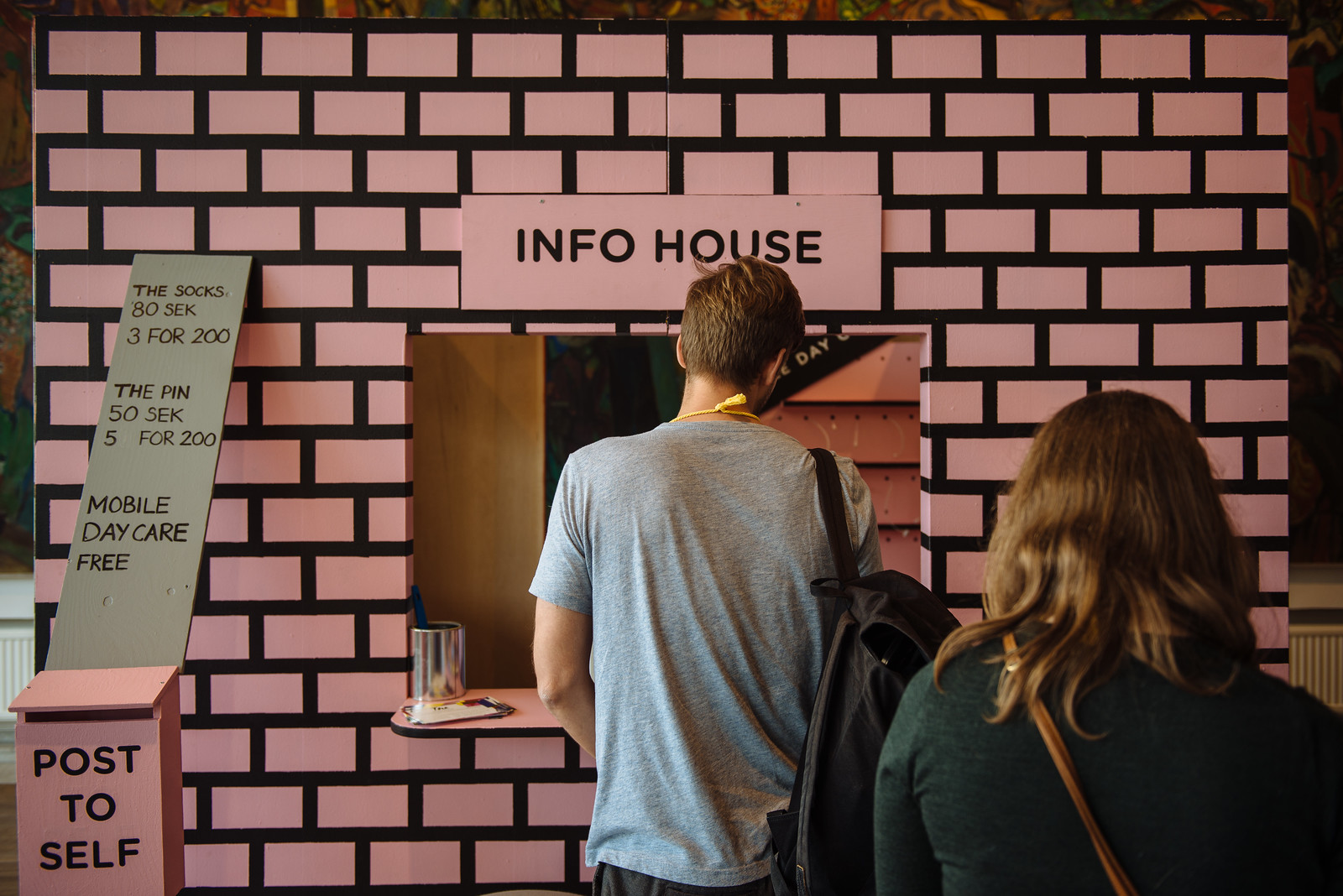This photograph showcases a whimsical, makeshift "Info House" with a facade resembling white bricks on a black grout, seemingly constructed from cardboard or particle board. At the center of the facade is a service window with the label "Info House" above it, suggesting a place where services or items can be requested or purchased. To the left of the window, multiple signs are displayed: "The socks 80 sec, 3 for 200," "The pin 50 sec, 5 for 200," and "Mobile daycare free." Additionally, there is a small mailbox labeled "Post to Self." In front of the window, a line of people with backpacks waits, with a man in a gray t-shirt and black backpack currently at the counter and a woman with a gray or green sweater, brown hair, and a brown leather purse behind him. The setting appears to be a creative, pop-up stand potentially for safekeeping personal items or providing information and services.